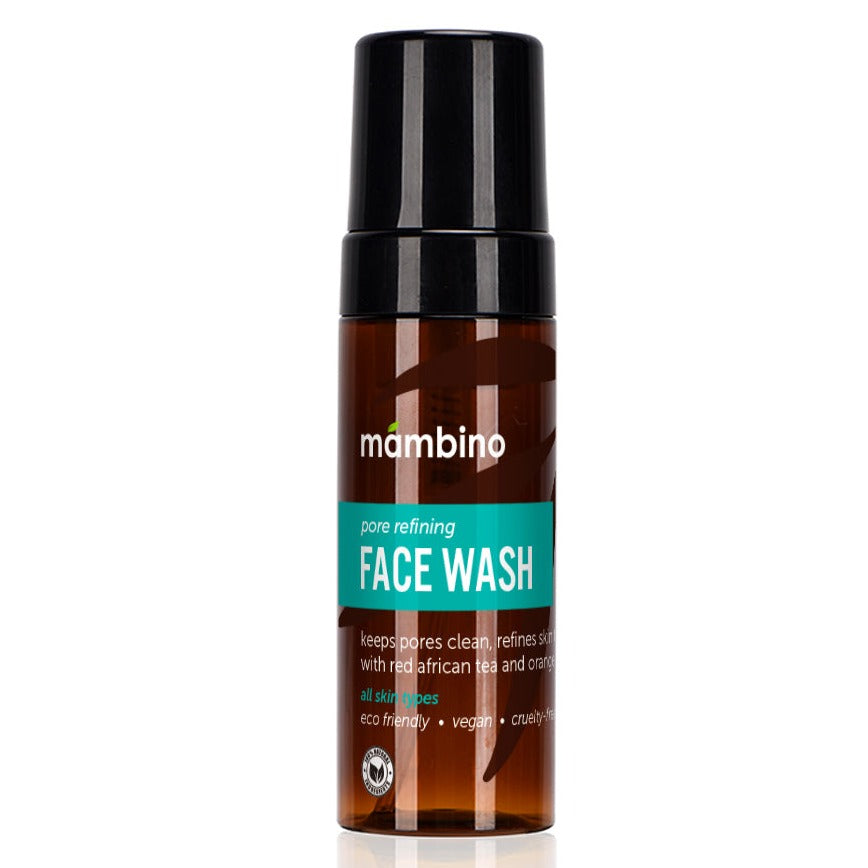The image depicts a small bottle, approximately three to four inches tall, filled with a dark cocoa-colored liquid. This product is a pore refining face wash by Mambino. The bottle, which appears to be made of either glass or plastic, features a transparent section allowing the brownish liquid inside to be visible. The bottle is topped with a black twist-off cap.

On the bottle, an aqua-colored band runs across the middle, displaying "Pore Refining Face Wash" in large white font. Additionally, smaller white text reads "Keeps Pores Clean, Refreshes with Red African Tea and Orange." The text "All Skin Types" is highlighted in aqua, while further down, you can see the words "Eco-Friendly, Vegan, Cruelty-Free" also in white font. 

The brand name "Mambino" is prominently displayed at the top in white letters, with a distinctive green leaf icon positioned above the 'M'. A certification logo is present on the lower left-hand part of the bottle. This detailed presentation emphasizes the product's key features and eco-friendly credentials.